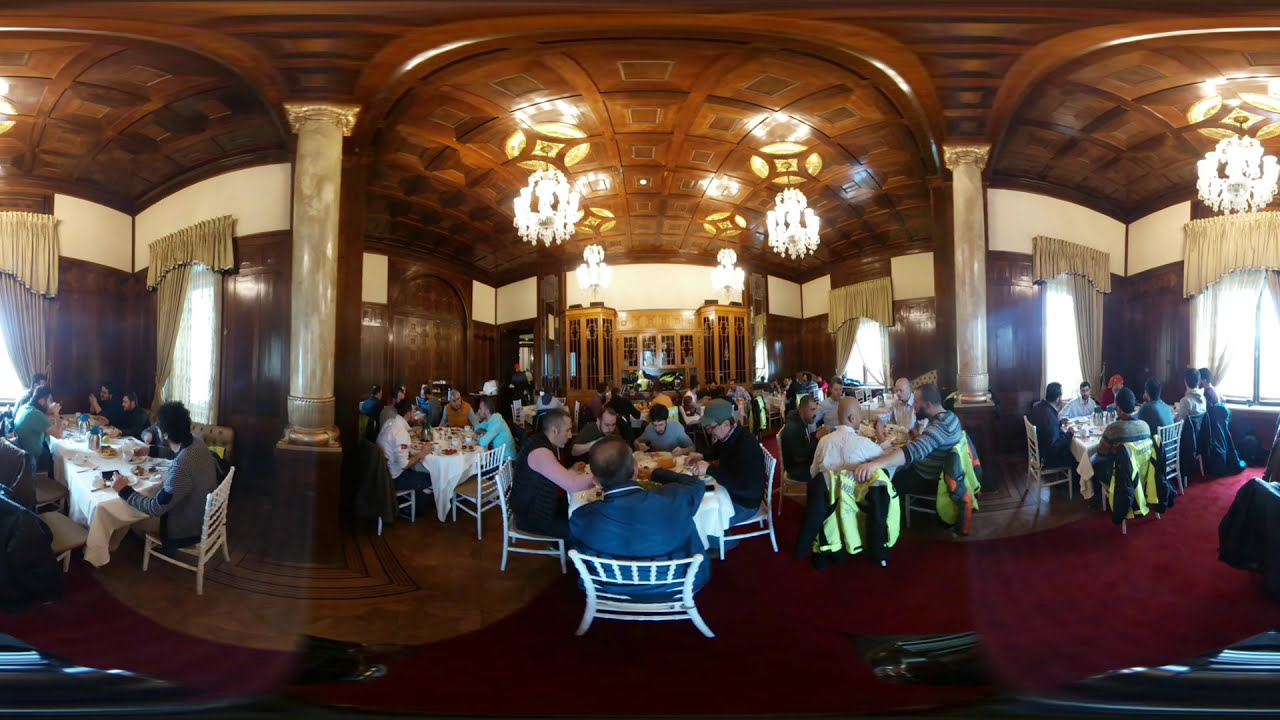This image captures an elegant indoor gathering, likely in a high-end restaurant or part of a hotel. The setting features multiple round and square tables adorned with white tablecloths and surrounded by white chairs, all of which are occupied by people enjoying a meal. The room is lavishly decorated, with ornate chandeliers hanging from a complex, brown wood ceiling accented by long, intricate pillars. Cream-colored curtains frame the tall windows on both sides, allowing daylight to flood in and illuminate the space. The flooring is an interesting mix of red carpet and brown wood, with some exposed tile areas. In the background, a large wooden cabinet and a set of doors are visible. The photograph itself has a fisheye or panoramic effect, creating a slightly warped, rounded perspective that emphasizes the room’s grandeur and the full, busy atmosphere.